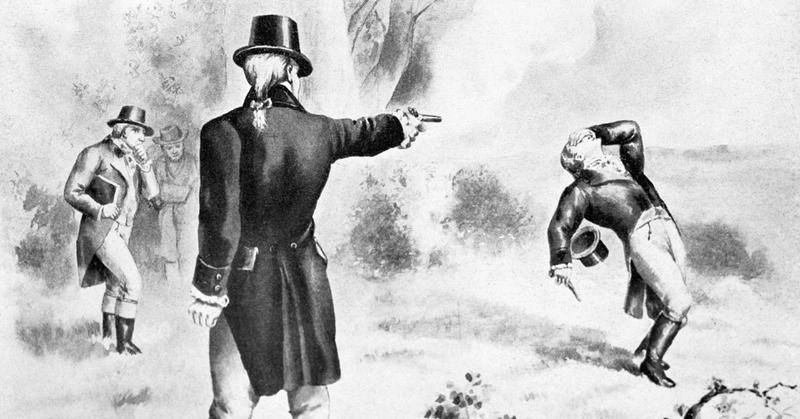This is a detailed black and white illustration depicting a dramatic duel scene likely set in colonial times. The central focus is a man in an overcoat and top hat with a white ponytail, who is pointing a pistol at another man who is falling backward, his hat toppling off. The fallen man, clad in similar attire—trousers, calf-high boots, and an overcoat—seems to be clutching his face in agony. The confrontation is being observed by two other men. One on the left, appearing contemplative with a hand under his chin and a book under his arm, is dressed similarly in a top hat and overcoat. The second observer stands near a tree, wearing a regular hat, closely watching the intense moment from a distance. This masterfully captures the moment of a pistol duel with striking period details and emotive expressions.